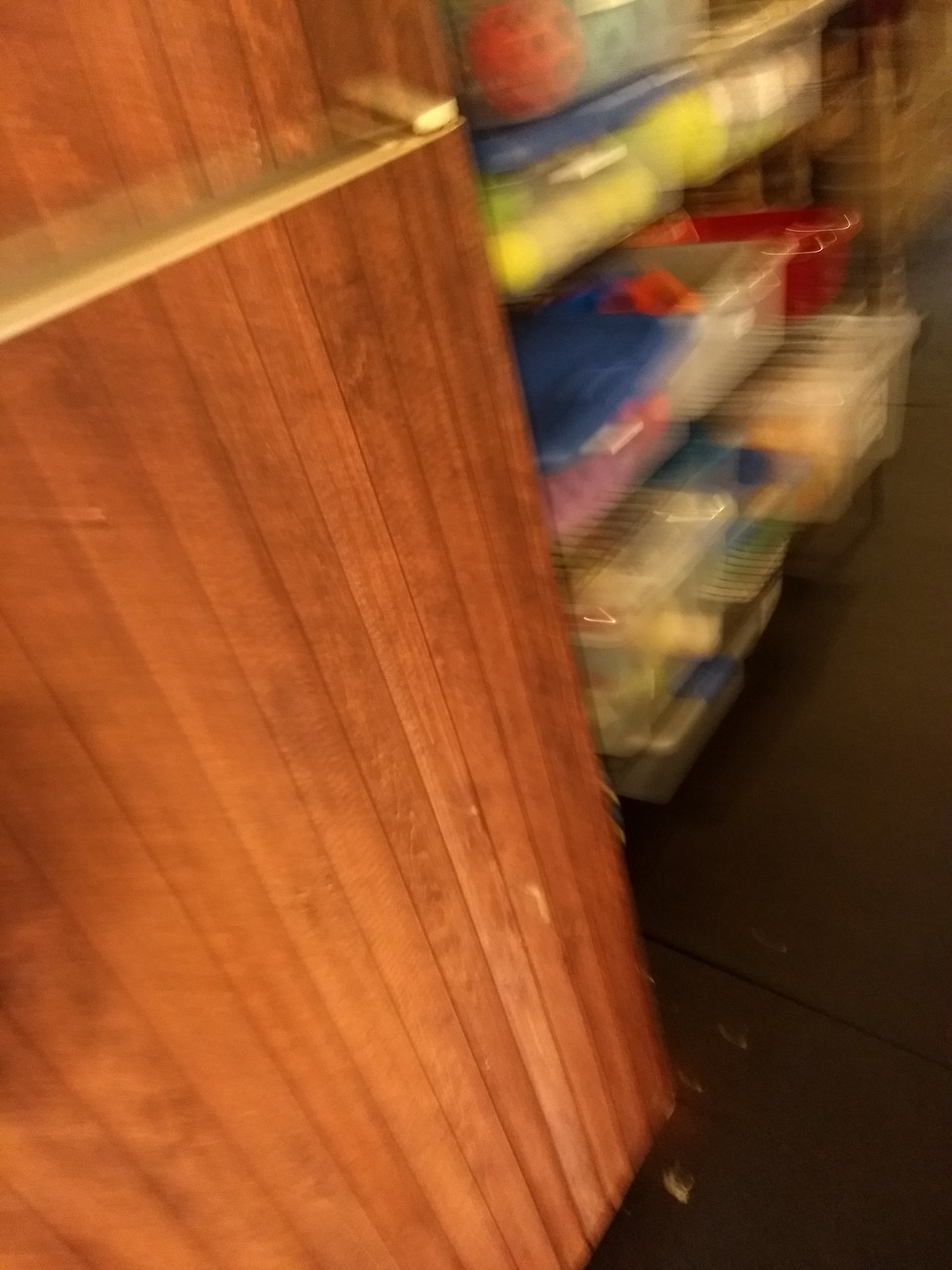This vertical, rectangular image captures the interior of what appears to be a closet within a home. The closet floor, though indistinguishable between wood or carpet due to its dark, chocolate brown hue, forms a stark foundation. To the left, a door or wall made of narrow wood planks is visible, featuring a brass bar handle. The image's significant blurriness gives it a surreal, double-vision effect.

The closet interior features wire shelves stocked with an organized array of containers. Four shelves are discernible: the lowest shelf holds a clear container to the right, flanked by a small clear container with a blue lid in the center, and another larger clear container adjacent to it. The second shelf from the bottom also holds three containers, while the third shelf appears to have another row of about three containers, all shrouded in the same blur. The closet's background is lined with another set of wood planks, darker in tone, displaying a blend of black and brown colors, complementing the overall composition.